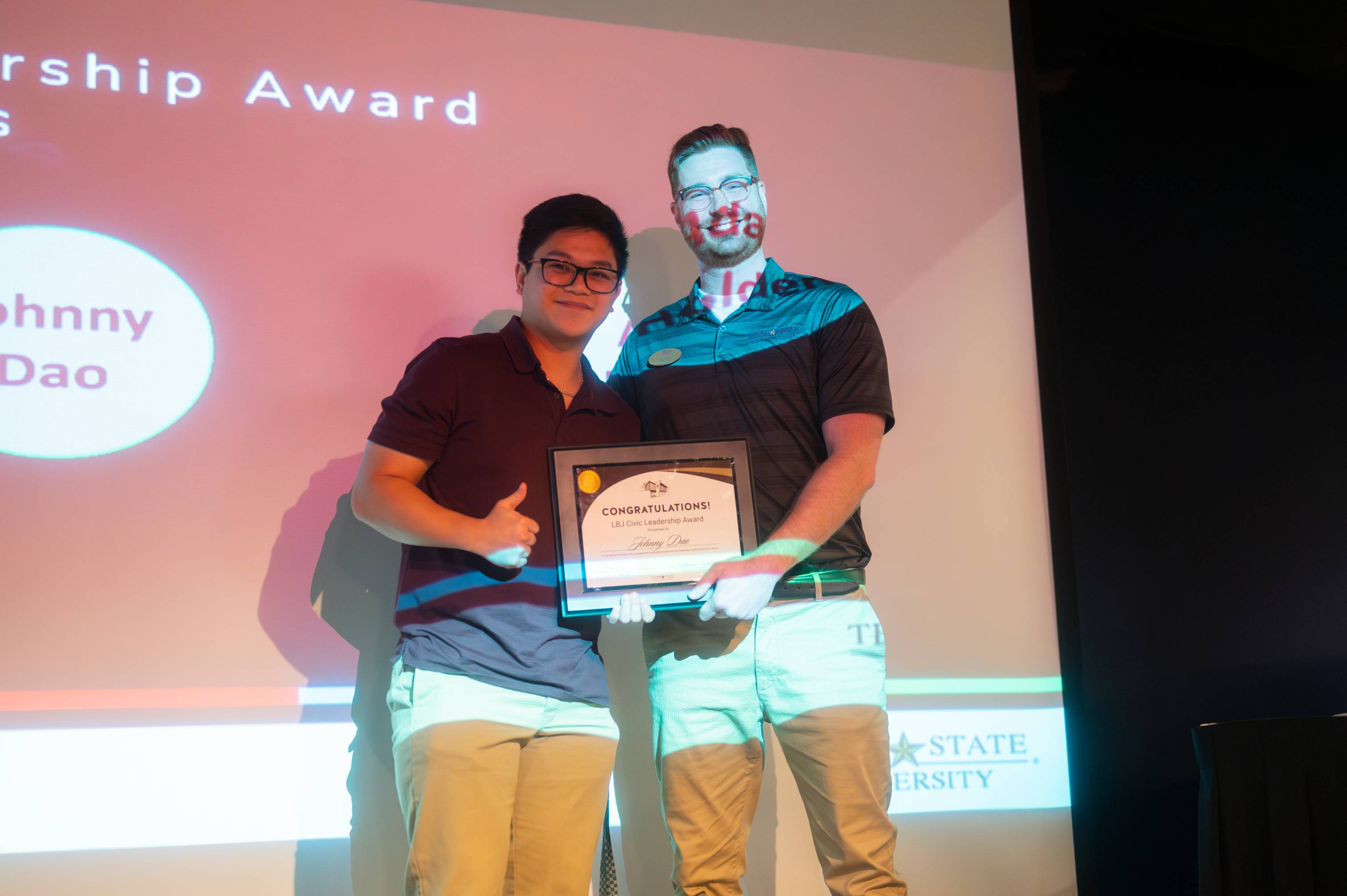The rectangular image captures a moment on stage featuring two individuals who are likely at a university event. On the right stands a slightly older Asian man with thick glasses, wearing a brown-collared, short-sleeve golf shirt and tan khaki pants. To his left is a younger, taller white boy with thin glasses, dressed similarly in a brown golf-style collared shirt and tan khaki pants. Both individuals are holding a plaque together, suggesting it is an award, most likely won by the younger boy, who's giving a thumbs-up gesture. Behind them is a large screen projecting a slideshow that partially reveals the words "AWARD" and "SHIP," implying it might be a Leadership Award. There are fragmented words like "HNNY" and "DOE," possibly part of the recipient’s name or the person the award is named after. Additionally, "State University" is visible at the bottom, indicating the venue, though the exact name is cut off. The projector light casts an image onto the screen and partially onto the older man's face, creating an unusual effect.